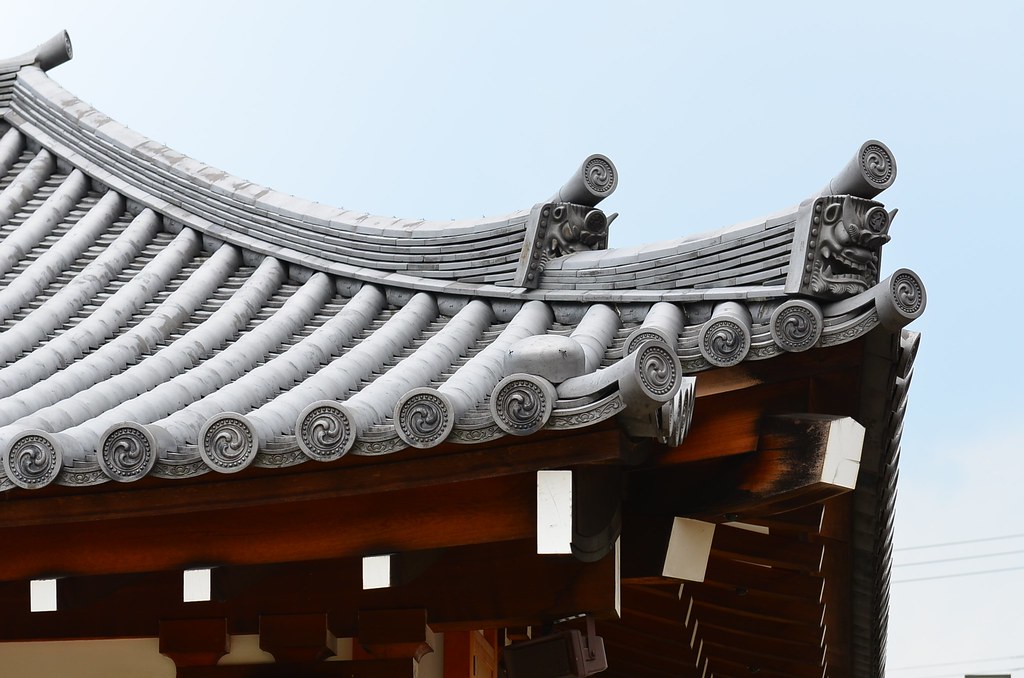This detailed photograph captures a captivating corner of East Asian architecture, possibly from a Japanese temple, set against a clear, pale blue sky. The roof, composed of meticulously hand-crafted gray tiles, slopes from the top left to the center of the frame, featuring smaller, similar slopes beneath it. Decorative gray tubes extend from the edges of these slopes, each capped by ornate, intimidating dragon heads that add a sense of fierce elegance to the structure. Beneath the roof, rows of gray tubes create a flowing pattern across the main gray ridged surface. Supporting this architectural marvel are tall and wide red wooden beams, adorned with bright white rectangular caps, offering a striking contrast against the subtle hues of the roof. The lower portion reveals a beige wall, adding depth and dimension to the scene. In the background, a set of five power lines, three above and two below, stretch across the sky, blending modern elements with traditional craftsmanship.